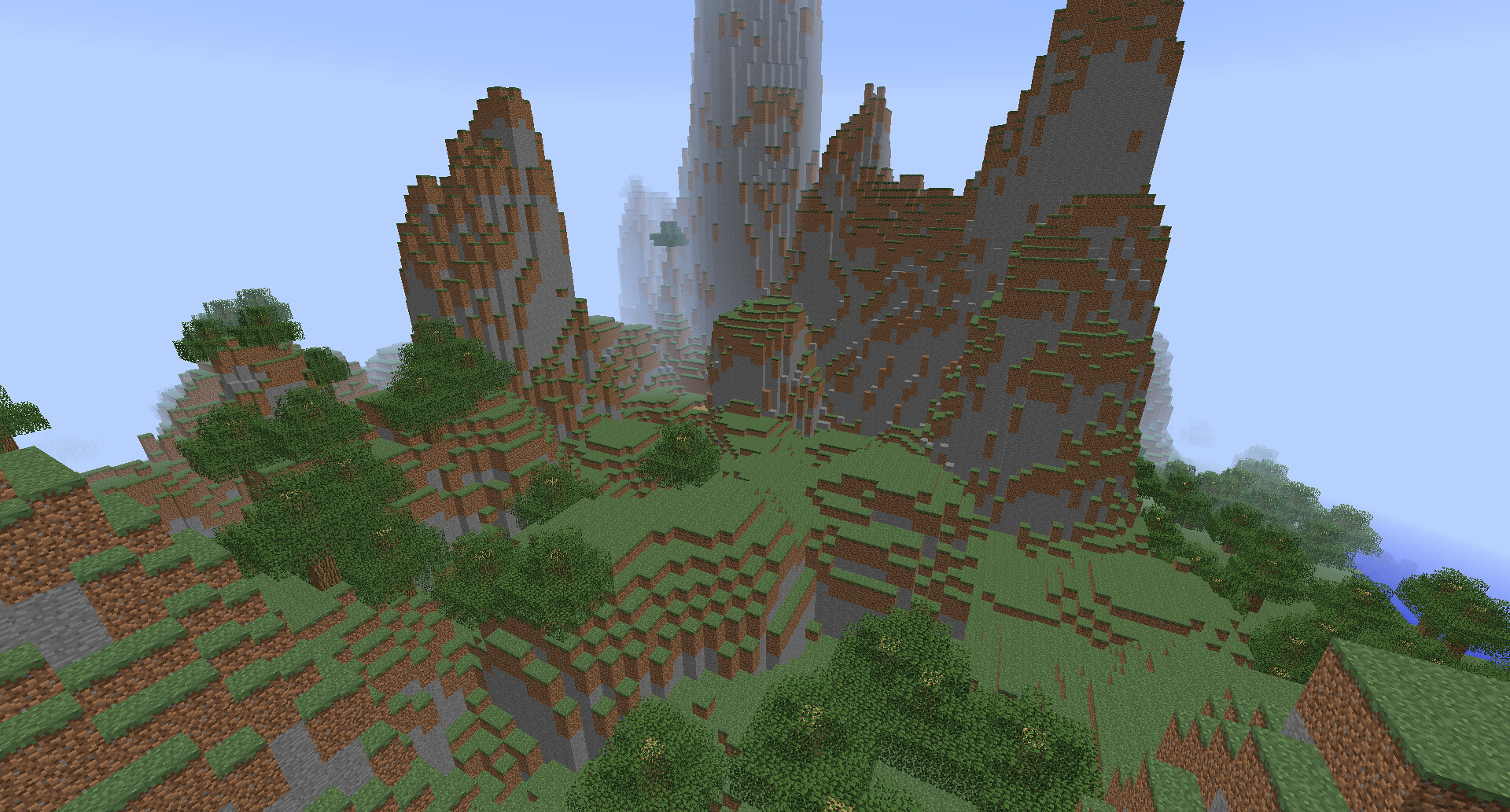This image appears to be a screenshot from the video game Minecraft, captured from an aerial perspective. The scene depicts a rugged mountain landscape with several gray stone mountains, interspersed with patches of brown earth topped with lush green vegetation. Specifically, three distinct mountains can be identified, surrounded by areas dense with various types of bushes and plant life. The sky above is a clear, bright blue, indicating that the scene is set during the daytime within the game. The overall composition showcases the game's characteristic blocky, pixelated graphics, giving a sense of depth and texture to the natural environment.